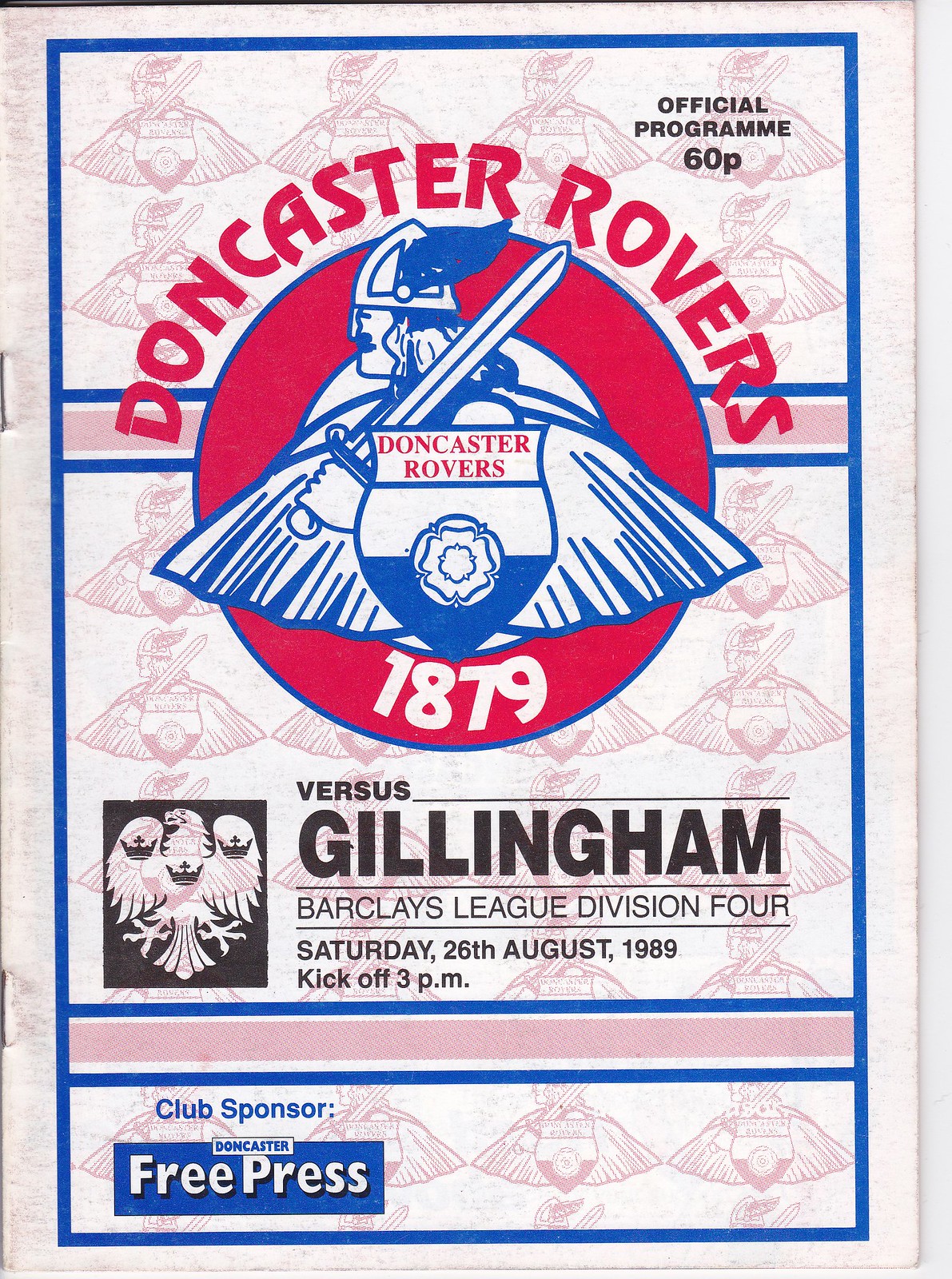The image is the front cover of a magazine or brochure, predominantly featuring a repeating background pattern of a Viking logo in light red against a white backdrop. Central to the design is a cartoonish Viking figure with a winged helmet, blue and white cape resembling bat wings, and carrying a sword and shield. The shield prominently displays the text "Doncaster Rovers" in red. Encircling this central figure is a large red ring with "Doncaster Rovers" written in bold red letters. At the top right corner of the cover, the text "Official Program 60P" appears in black. Inside the central shield, the year "1879" is noted in white.

Beneath the red circle, the text reads: "Versus Gillingham, Barclays League Division Four, Saturday, 26th August 1989, kick off 3 p.m." To the lower left corner, it states "Club Sponsor: Doncaster Free Press" with "Club Sponsor" in blue and "Free Press" in white, set against a blue rectangle. The entire cover is framed by a substantial blue border, adding to the overall striking and cohesive design of the page.